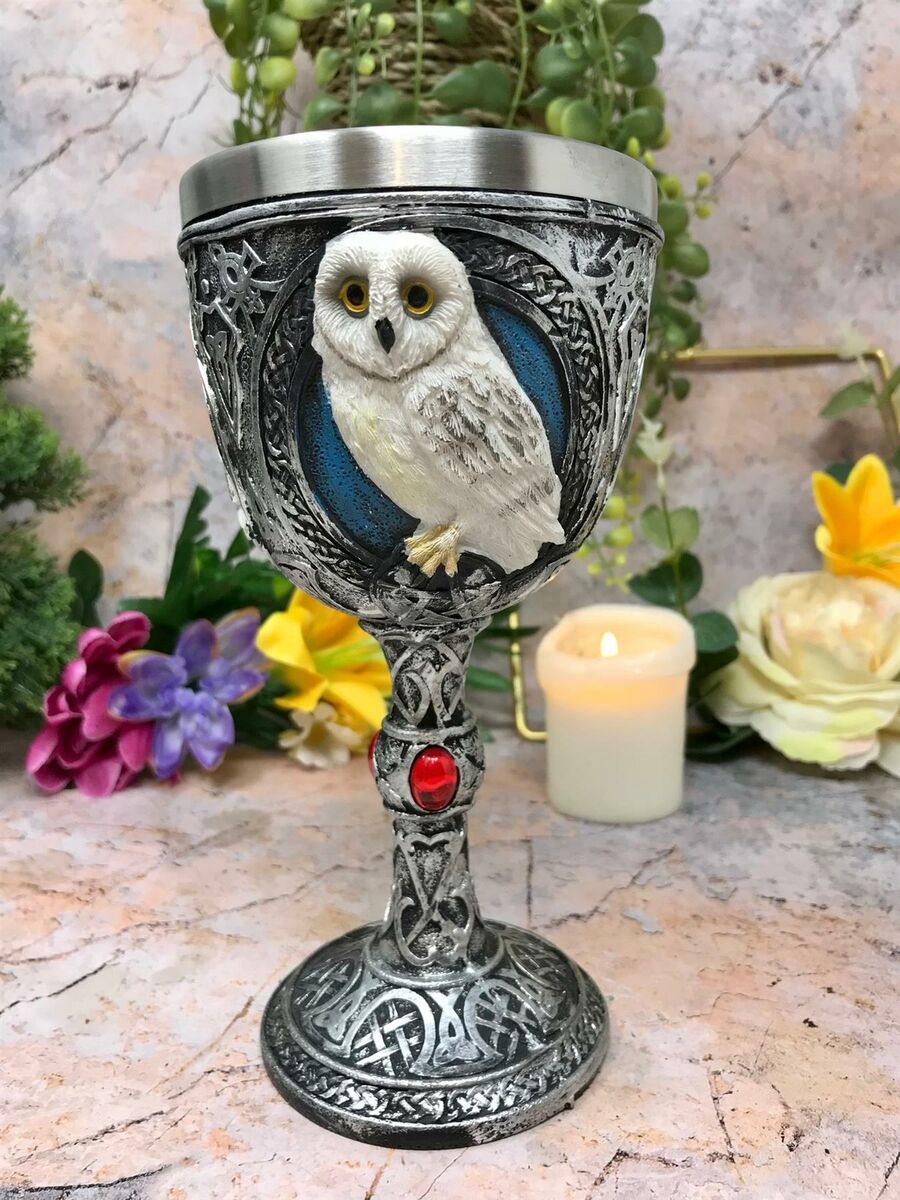In the center of the photograph, a meticulously detailed gothic-fantasy style goblet is perched atop a stone step. This pewter-toned goblet, designed to resemble aged silver, showcases an intricate Celtic design with crisscrossing, weaving patterns that flow from the base to the stem and around the bowl. Adorned with small red stones, the stem features a bulging section that enhances its ornate appearance. At the top of the goblet, an intricately sculpted white owl with gold rings around its translucent yellow eyes, a black beak, and yellow claws, is set against a blue-teal backdrop. The owl’s finely detailed feathers and lifelike appearance add a mystical quality to the goblet. Surrounding the goblet, the scene is framed by an array of colorful flowers, green foliage, and a lit cream-colored candle, creating an atmosphere reminiscent of a medieval fair or a fantasy ritual setting. Hues of blues, whites, yellows, pinks, violets, greens, and browns complement the metallic silver of the goblet, adding to the enchanting and immersive aesthetic of the image.